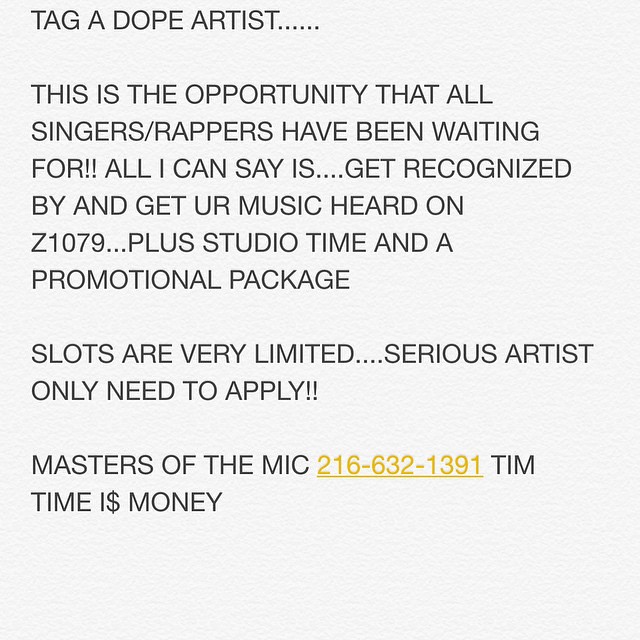The image features a screenshot of a notepad on a mobile device, with a light gray to blue background and predominantly black, all-caps text. The message urges viewers to "Tag a Dope Artist," emphasizing an unparalleled opportunity for singers and rappers to get discovered. It reads, "This is the opportunity that all singers/rappers have been waiting for!! All I can say is... get recognized by and get your music heard on Z107.9, plus studio time and a promotional package. Slots are very limited.... serious artists only need to apply!!" The slogan "Masters of the MIC" is prominently displayed, followed by the contact number "216-632-1391" in underlined gold text, along with the phrase "Tim Time is $ Money." The text occupies the entire screen, highlighting the potential benefits and exclusivity of this music promotion opportunity.